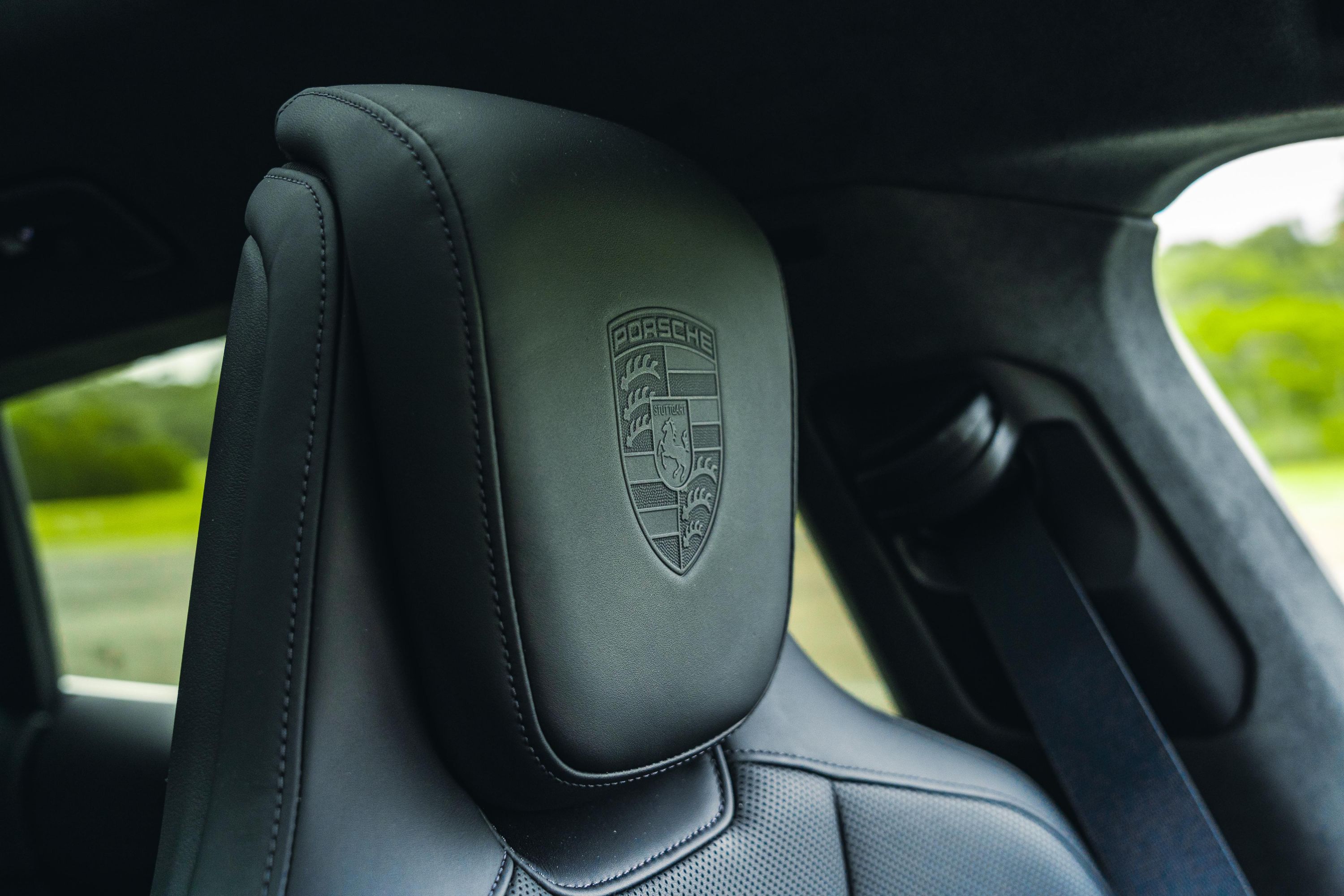This detailed close-up photograph captures the luxurious interior of a Porsche, focusing on the driver's seat headrest. The headrest is upholstered in dark gray leather with prominent stitching marks that give it a racing seat appearance. Dominating the center of the image, the headrest is slightly angled to the right, showcasing the meticulously embedded Porsche emblem, with "Porsche" elegantly inscribed above it. The photograph, framed in a horizontal rectangle and positioned just left of center, also reveals a seatbelt draped to the right of the headrest, extending off the image to the bottom right corner. Through the car windows in the background, a serene exterior with green trees and grass can be seen, suggesting the car is parked in a secluded, verdant area. The overall interior of the car is predominantly black, enhancing the sleek and sophisticated aesthetic.